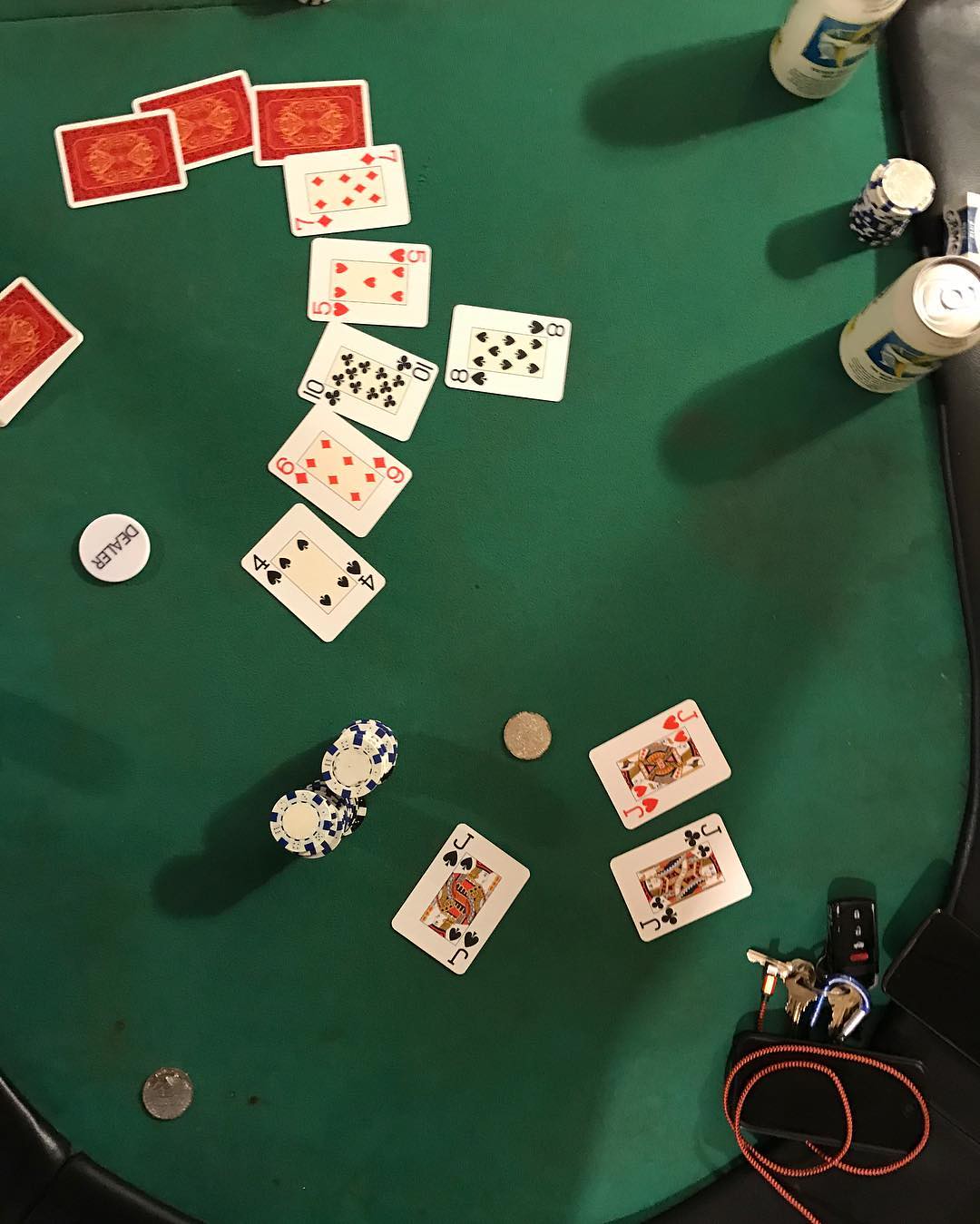This photograph captures a classic game night setting on a dark green card table, accentuated by a slightly raised black rim around the edges. The table, commonly used for poker or card games, is sprinkled with a mix of gaming paraphernalia and personal items. 

On the top right corner, two tallboy cans of beer stand unopened, suggesting a pause in the action for refreshments. Scattered across the table are several red playing cards, displaying a variety of ranks including the four of spades, six of diamonds, ten of clubs, five of hearts, seven of diamonds, and eight of spades. Three different jacks are prominently visible amid the spread.

In addition to the chaos of the cards, there are stacks of poker chips in various denominations and colors, alongside a few loose coins. The bottom right of the table features a clutter of personal items including a set of headphones and car keys. Adding to the authenticity of the gaming scene, a white chip marked "DEALER" in black text lies conspicuously on the table.

The dim lighting casts shadows over the objects, hinting at a late-night setting filled with the anticipation and strategy inherent to a card game in progress.